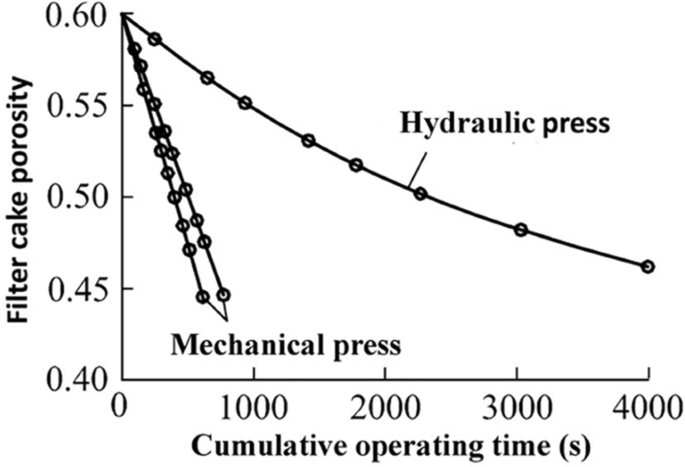This is a black-and-white graph displaying the relationship between filter cake porosity and cumulative operating time. The y-axis is labeled "Filter Cake Porosity" and ranges from 0.40 to 0.60, while the x-axis is labeled "Cumulative Operating Time" and ranges from 0 to 4,000. The graph features multiple lines: 

1. The primary line, labeled "Hydraulic Press," begins at a porosity of 0.60 and gradually slopes downward to a porosity closer to 0.40 by the time it reaches a cumulative operating time of 4,000.
   
2. There are two additional lines, steeper in decline, labeled "Mechanical Press." These lines also originate from the upper section of the y-axis but converge around the 1,000 mark on the x-axis, indicating a sharper decrease in porosity over a shorter period.

The graph's background is completely white, enhancing the clarity of the plotted lines and labels.